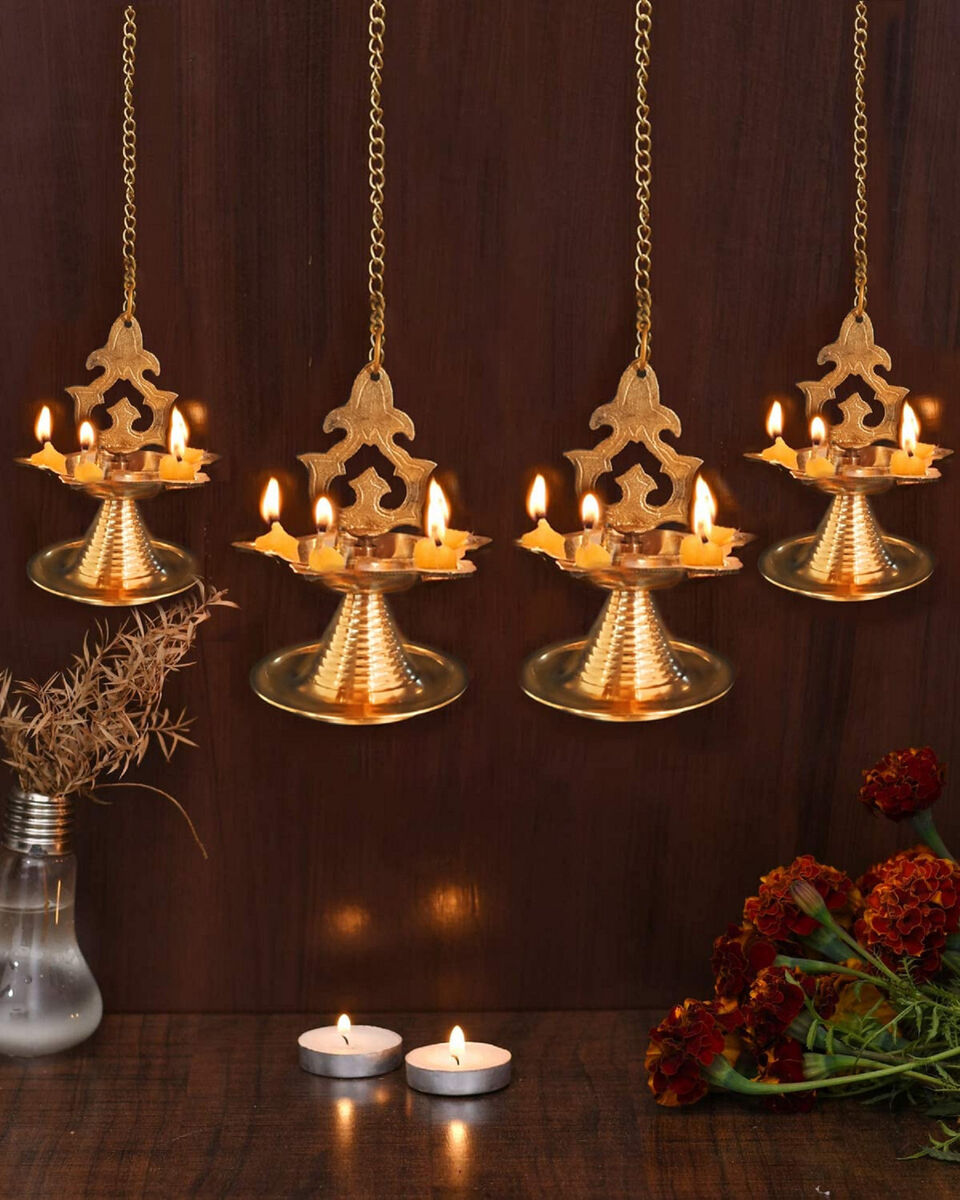The image features a shiny brown wooden table at the bottom, adorned with two small, lit disc-like candles encased in silver dishes positioned next to each other. To the left of these candles, there’s an upside-down light bulb filled with water, from which dead plants are protruding. On the right, vibrant green stems with circular clusters of small red flowers are arranged. In the background, four gold-colored candle holders with a spiral handle design and a small platform hold glowing candles. The candle holders are mounted on a wooden partition wall, with decorative gold chains extending from it. Hanging from these chains are small wax piles with string wicks, forming unique candle arrangements, adding a layered depth to the scene.